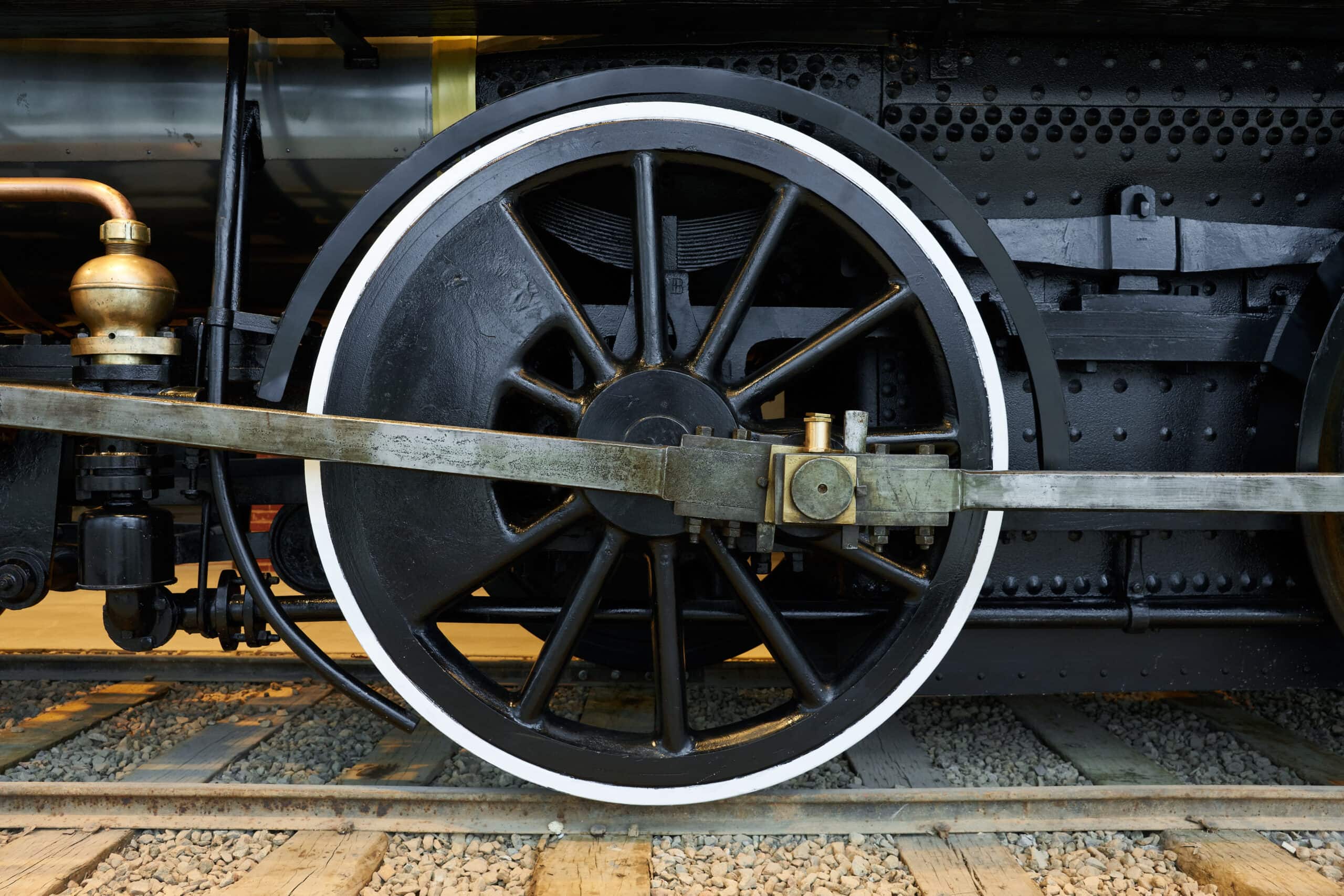This detailed close-up image showcases the underbelly of an old locomotive, specifically focusing on a large jet black train wheel with matte black spokes radiating from its center and a distinctive white rim encircling it. The wheel is central in the frame and prominently displays its mechanical intricacies. Attached to the wheel are metal rods, a brushed silver in appearance, running horizontally across the image. 

To the left side, a golden copper piston, part of a complex mechanical system of black tubes and a metal bar, aids in the wheel's rotation. The locomotive's casing is also a deep black and exhibits a series of raised circular features extending from top to bottom on the right side of the image.

The train rests on light brown wooden beams, weathered with cracks and splintering, embedded in a bed of silver and gray gravel, a stark contrast to the rusty, dusty metal tracks they support. The entire scene exudes a sense of stillness, evoking a bygone era of rail travel.